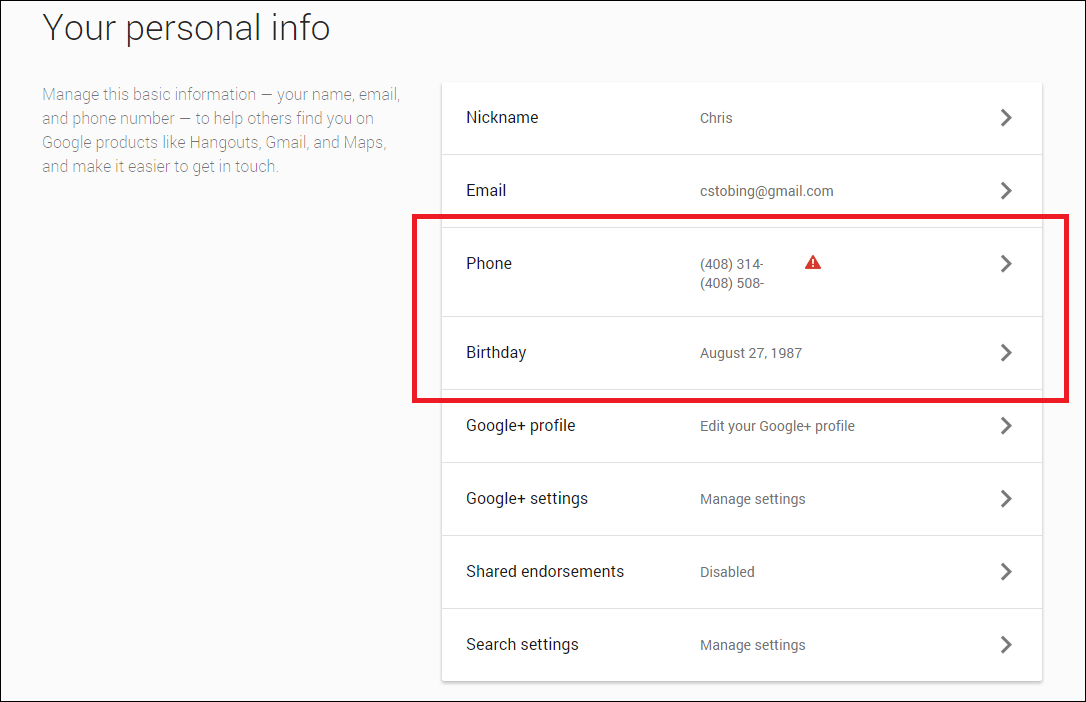The image depicts a simple black and white webpage designed for managing personal information for Google products. At the top, there is a header titled "Personal Info," which includes basic details such as name, email, and phone number. These details are intended to help others find Google products like Hangouts. To the right of the personal information section, there is a nickname field currently displaying "Chris," which can be edited. Beneath this is a right arrow icon.

Further down, there’s an email list featuring "cs2bing, cs2bing@gmail.com," followed by an incomplete phone number that shows only the area code and the first three digits. The birthday listed is August 27, 1987. Below these details is a link to edit the Google Plus profile.

Continuing further, there are settings sections labeled "Google Shared Endorsements" and "Search Settings," where users can manage their visibility and interaction preferences for a more personalized Google experience.